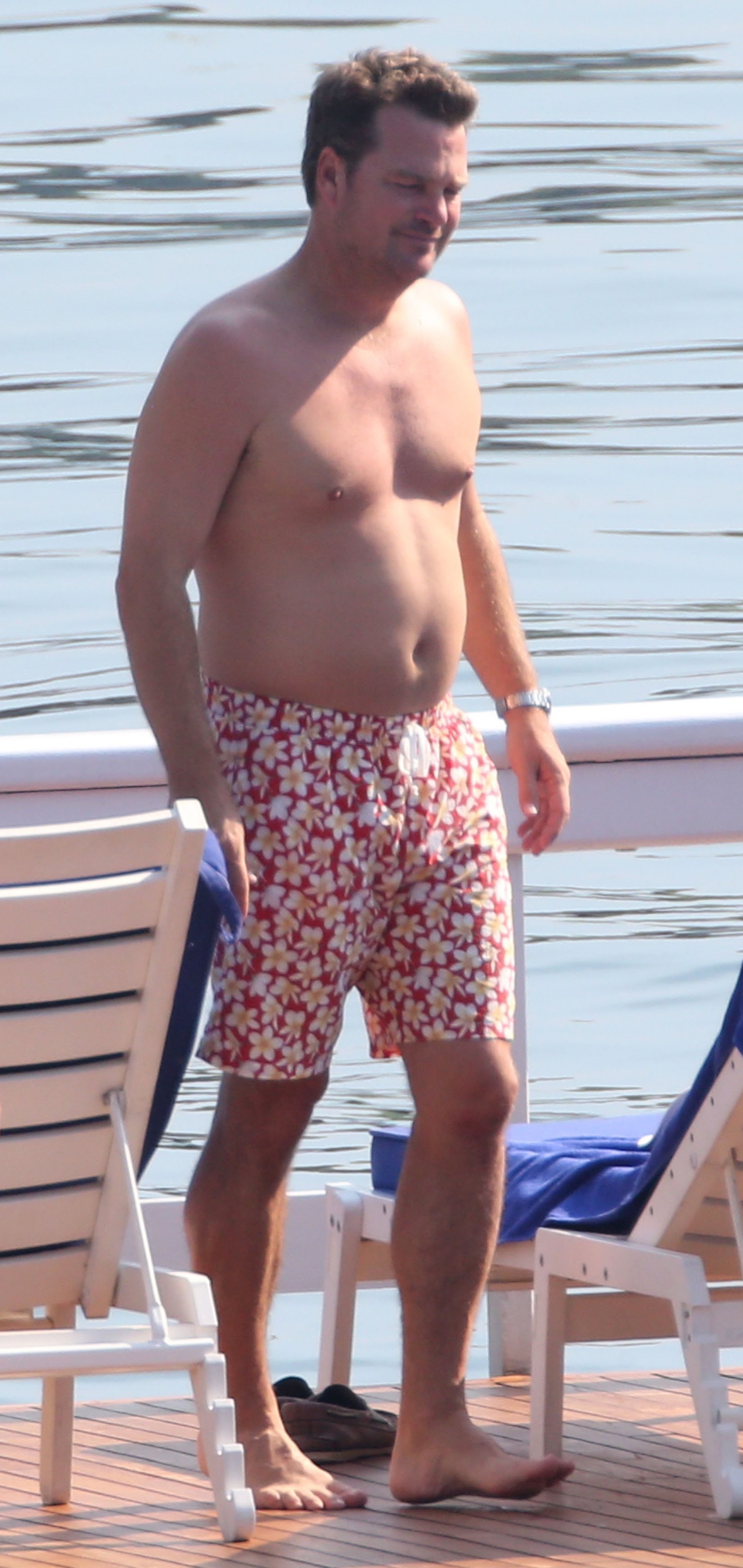This outdoor photograph captures a shirtless, slightly older man with short dark hair and a bit of stubble, standing barefoot on a wooden deck. He is wearing red swim trunks adorned with a pattern of white and yellow five-petaled flowers and a silver watch on his left wrist. The deck, made of tan-colored wood, is part of a boat, highlighted by a waist-high, stark white railing behind him. Flanking him are two white wooden lounge chairs, one draped with a blue towel and another covered in a cushion with a blue pad. Dark gray shoes with white stripes along the soles are positioned near him. In the background, a calm, clear body of water stretches out, reflecting a cloudy sky, creating a serene and tranquil scene.